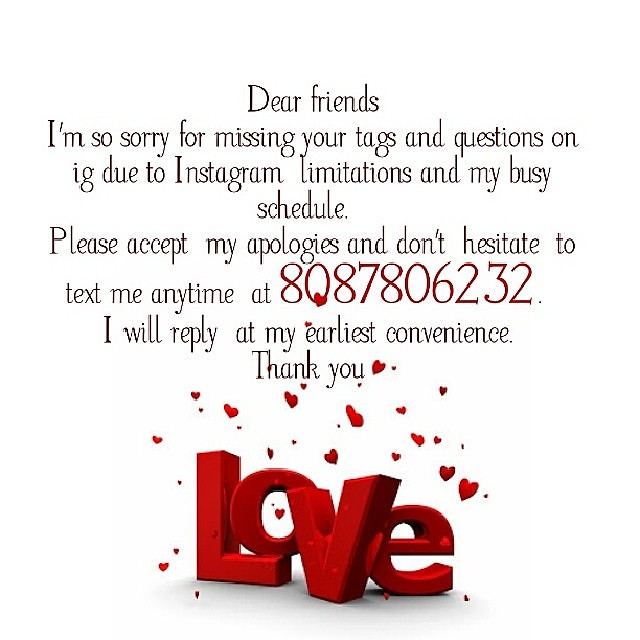The image is a white-background screenshot of an Instagram post that serves as both an advertisement and a thank-you note. The central text, written in a black script, reads: "Dear friends, I'm so sorry for missing your tags and questions on IG due to Instagram limitations and my busy schedule. Please accept my apologies and don't hesitate to text me anytime at 8087-806232. I will reply at my earliest convenience. Thank you." The phone number is highlighted in red text. Below this message, a large, centrally located graphic features a 3D representation of the word "love" in red, with the letters artistically arranged— the 'O' balancing on the 'L,' the 'V' pointing forward, and the 'E' positioned behind the 'V.' Scattered around the word are red hearts that resemble confetti, further emphasizing the theme of love and appreciation. Overall, the detailed design and color choices underscore a heartfelt attempt to connect with followers despite a busy schedule.